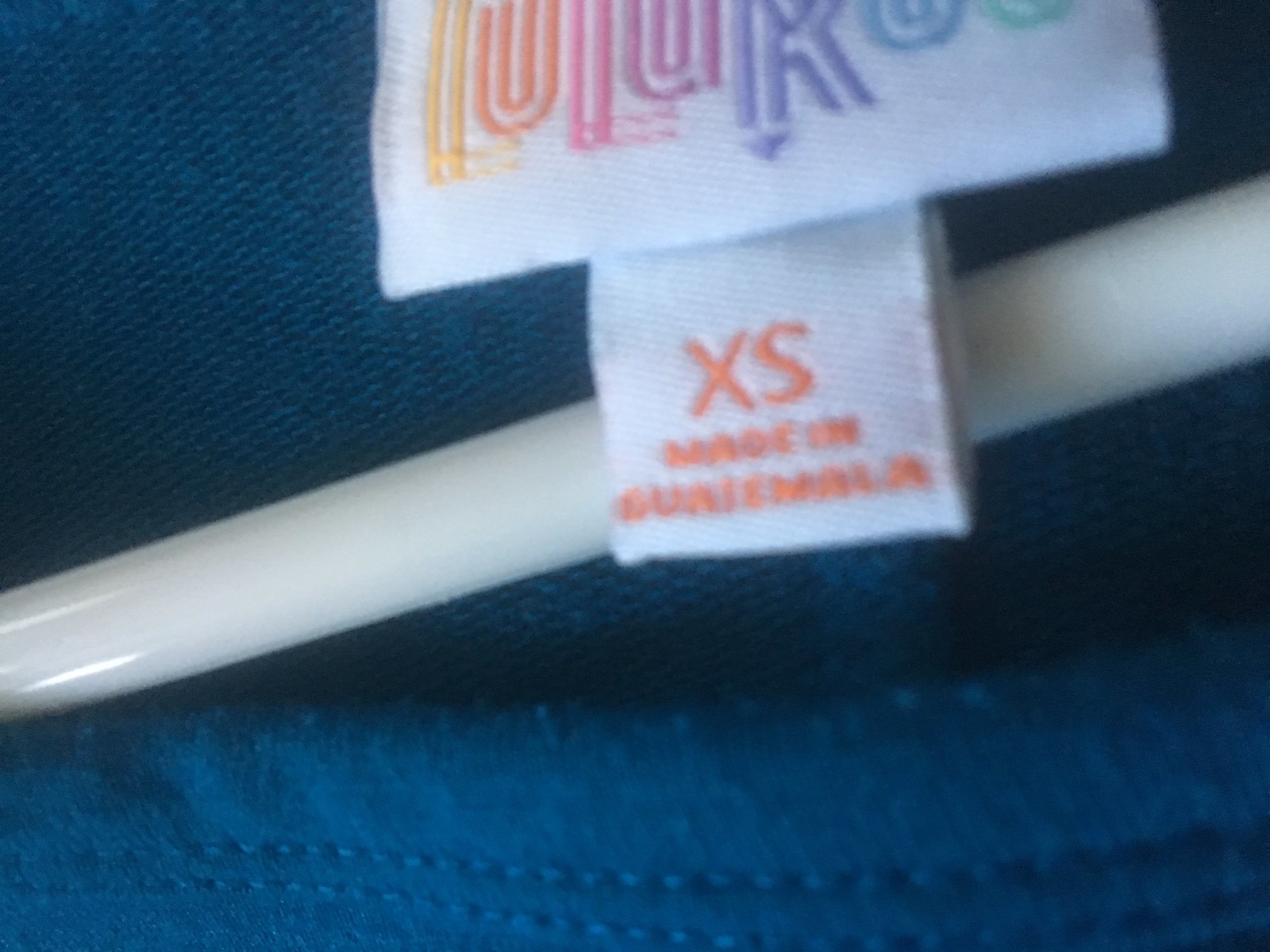This angled photograph captures the back of a shirt, focusing on its tagging detail. Centered in the frame is the shirt's large rectangular tag featuring the brand name "LuLaRoe" displayed in vibrant, colorful letters. Directly beneath it, a smaller square tag is fully visible, indicating the garment's size as "Extra Small." A white plastic rod, part of the coat hanger holding the shirt, is seen running diagonally from the bottom left to the top right of the image. The neckline of the shirt is partially visible at the bottom of the photo, revealing noticeable pilling with small fabric balls scattered on its surface, suggesting wear.